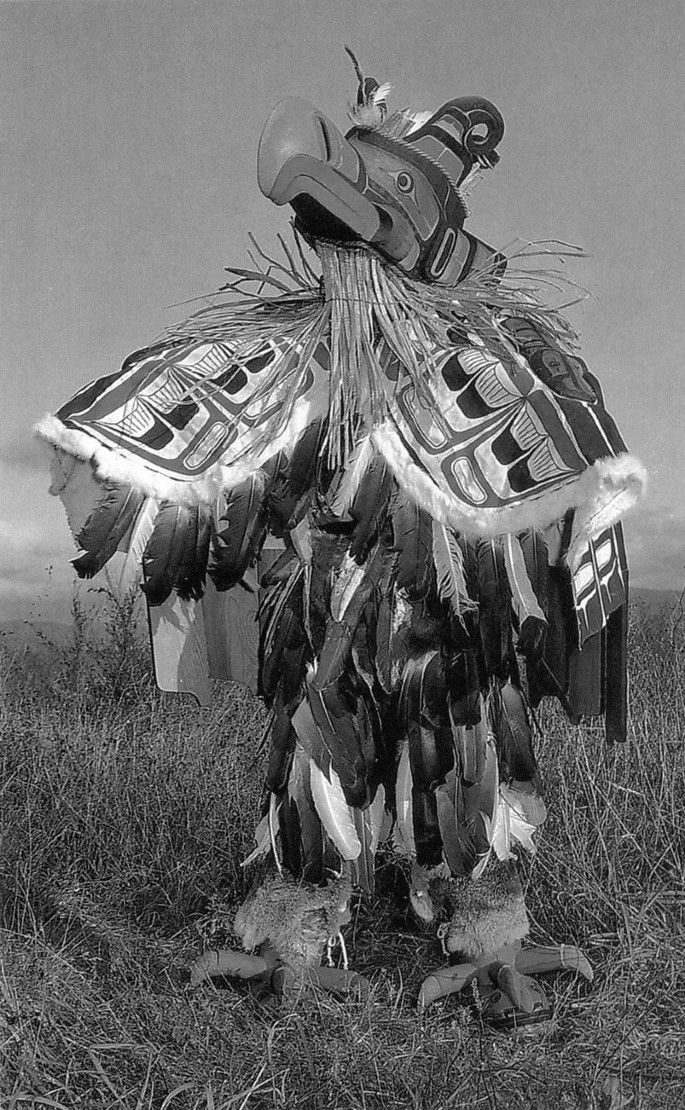In this detailed black-and-white photograph, a striking scarecrow-like figure stands prominently amidst tall, grassy plains. The figure resembles a hybrid between a Native American statue and a person dressed up as a bird, suggesting a cultural significance, possibly American Indian. Topped with an elaborate bird's head made of wood, with a long, extended beak and feathers adorning it, the headgear extends outward like wings. The head or hat also features a distinctive curled tip. The figure's shoulders are draped with a quilt-like cloak, under which countless feathers cascade down, enveloping the body entirely down to the exemplary chicken-like feet, each detailed with claw points. This avian figure is placed against a backdrop of endless gray haziness, with no visible sun or clouds, emphasizing the monochromatic essence of the photograph.